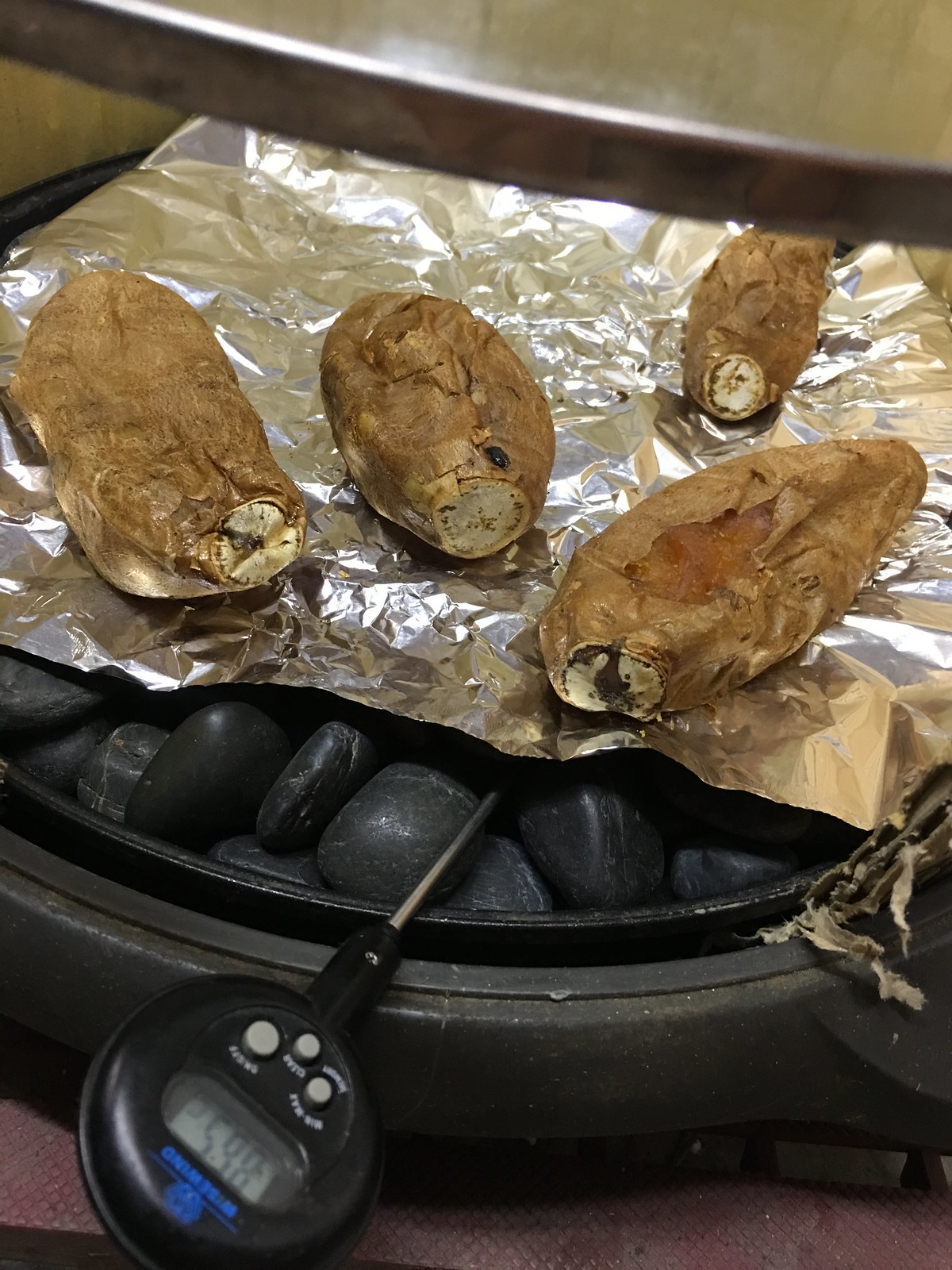The image depicts a somewhat unsettling scene of four brown, shriveled root vegetables, which appear to be Japanese sweet potatoes or possibly yuccas, placed on a piece of aluminum foil. The foil rests on a black grill or perhaps an electric frying pan, characterized by what seems to be black stones or a cast iron surface underneath. The vegetables are extremely overcooked, showcasing a dark brown color with splotches, giving them a rather unappetizing and gross appearance. A food thermometer, protruding from the foil and showing a reading of either 86.5 or 59.8 (the exact number is unclear), is also visible, though the brand cannot be discerned. The red textured surface below the grilling setup adds a contrasting background to the unsettling scene.